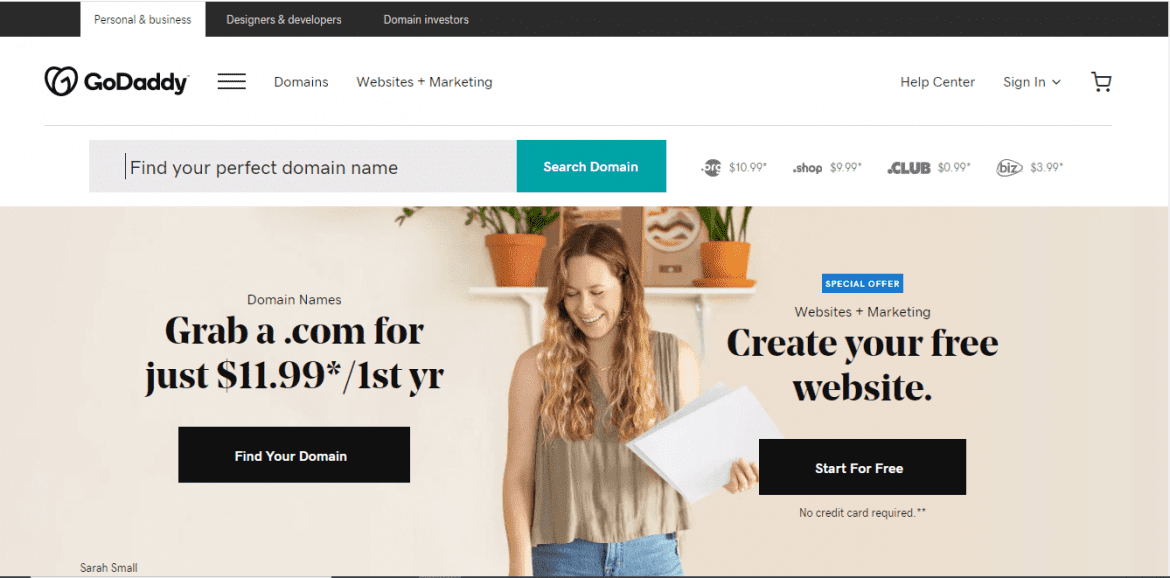This image is a detailed screenshot with a predominantly horizontal layout. At the very top, there is a solid black header featuring a white tab on the right side with black text that reads 'Personal', 'Business', 'Designers and Developers', and 'Domain Investors'. 

Directly below this header is a white banner showcasing the GoDaddy logo, which is heart-shaped and followed by the bold black text 'GoDaddy'. On the upper right corner of this white banner, there are options for 'Help Center', 'Sign In' with a dropdown arrow, and a shopping cart icon.

Beneath the white banner is a gray search bar where the placeholder text instructs users to 'Find your perfect domain name'. To the right of this search bar is a green action button labeled 'Search Domain'.

In the main section of the screenshot, there is a color photograph of a woman with long brown hair. She is casually dressed in jeans and a short-sleeved shirt. The woman is standing in a room and holding two pieces of white paper in her left hand.